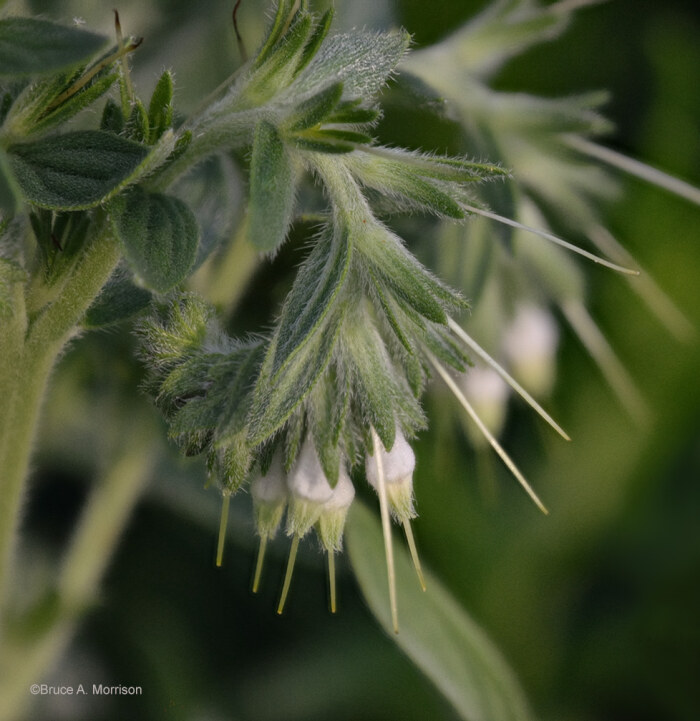The photograph, captured outside by Bruce A. Morrison (as indicated by a small, white copyright text in the bottom left corner), showcases a Sahari false gromwell plant, commonly seen in regions like Iowa or Montana. Dominating the left to center of the image is a tall, green, fuzzy stem adorned with flimsy, fur-covered leaves. These delicate leaves extend outward, supporting clusters of white flower buds that dangle downward. Each bud is accentuated by thin, straw-like structures protruding from its center. The background is a lush, green blur, featuring more of the same plant, adding depth and emphasizing the outdoor setting.